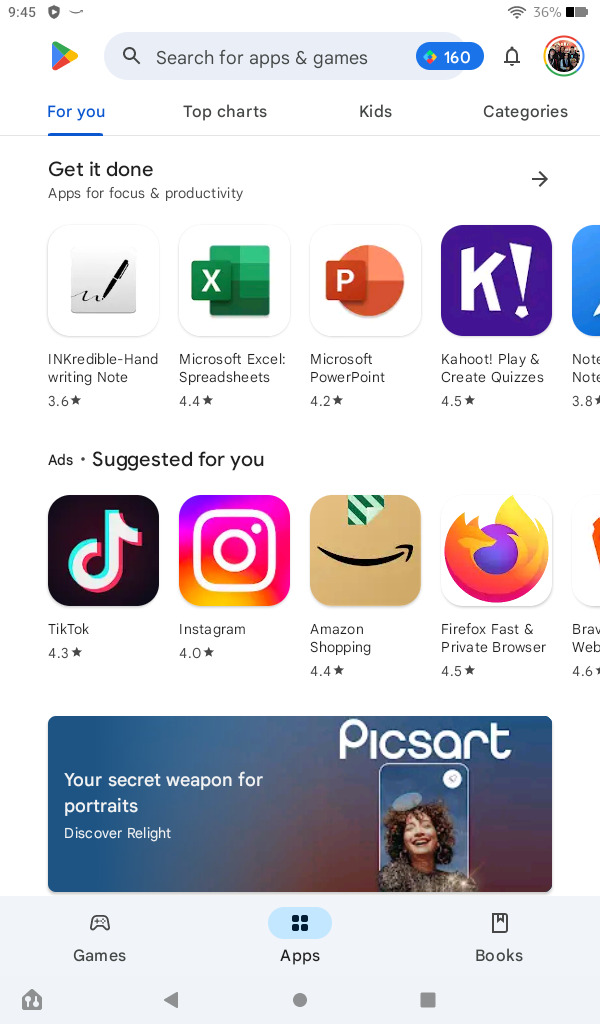This screenshot captures a typical view of the Google Play Store interface on a smartphone at 9:45 AM, with a 36% battery life remaining. Prominently at the top, the Google Play Store icon is displayed, composed of a multi-colored arrow segmented in green, blue, yellow, and red. The search bar suggests, "Search for apps and games."

Below the search bar, a diamond-shaped icon, also in green, blue, red, and yellow, is associated with the number "160." The navigation bar beneath it highlights various options: "For you" is underlined, emphasizing it as the currently selected category, alongside "Top charts," "Kids," and "Categories."

The section "Get it done. Apps for focus and productivity" features various applications like:
- "Ink: readable, handwriting note," rated 3.6 stars.
- "Microsoft Excel: spreadsheets," rated 4.4 stars.
- "Microsoft PowerPoint," rated 4.2 stars.
- "Kahoot: Play and Create quizzes," rated 4.5 stars.

Following these, a segment titled "Ads, suggested for you" showcases:
- "TikTok," rated 4.3 stars.
- "Instagram," rated 4 stars.
- "Amazon Shopping," rated 4.4 stars.
- "Firefox: Fast and Private Browser," rated 4.5 stars.

A highlighted blue oblong button with rounded edges reads, "Your secret weapon for portraits. Discover Relight." Off to the right, "PixArt" (spelled out in all caps as "P-I-C-S-A-R-T") is noted, accompanied by a photo of a smiling woman with curly hair.

At the bottom of the screenshot, the navigation options include "Games," "Apps" (which is currently selected), and "Books."